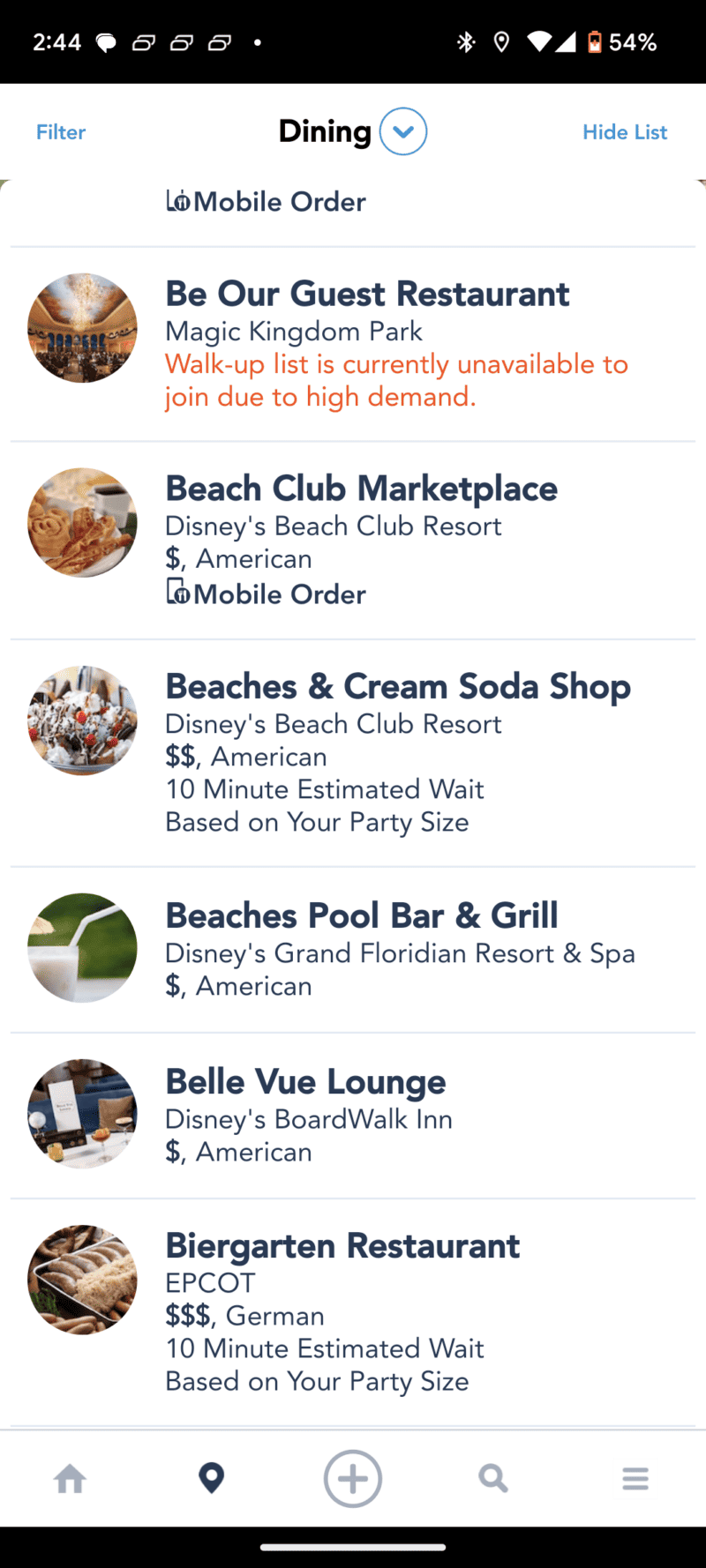In this vertically oriented smartphone screenshot from the Walt Disney app, various interface elements are clearly visible and informative. At the top, the black status bar shows essential phone information, including the time (2:44), Bluetooth connectivity, signal strength, a 54% battery level, and other icons.

Below the status bar, the main portion of the screen displays a clean white background. On the upper left, the word "FILTER" is highlighted in blue, while centrally positioned is "DINING," accompanied by a blue circle with an arrow for selecting additional options. On the upper right, "HIDE LIST" is visible.

The focal point of the screen is the "MOBILE ORDER" section under "DINING." This section features a series of circular icons, each representing a different restaurant with a corresponding image. Each listing provides the restaurant name in bold black text and its location within Walt Disney World Resort underneath. Among the options, "BE OUR GUEST" at Magic Kingdom Park is noted, with a message indicating that the walk-up list is presently unavailable due to high demand. Other locations listed include:

- Beach Club Marketplace at Disney's Beach Club Resort
- Beaches and Cream Soda Shop at the Beach Club Resort
- Beaches Pool Bar and Grill at Disney's Grand Floridian Resort
- Bellevue Lounge at Disney's Boardwalk Inn
- Beer Garden at Epcot

Some listings include dollar signs to indicate the price range of each dining option. At the bottom of the screenshot, various icons are visible, providing access to additional options and features within the app.